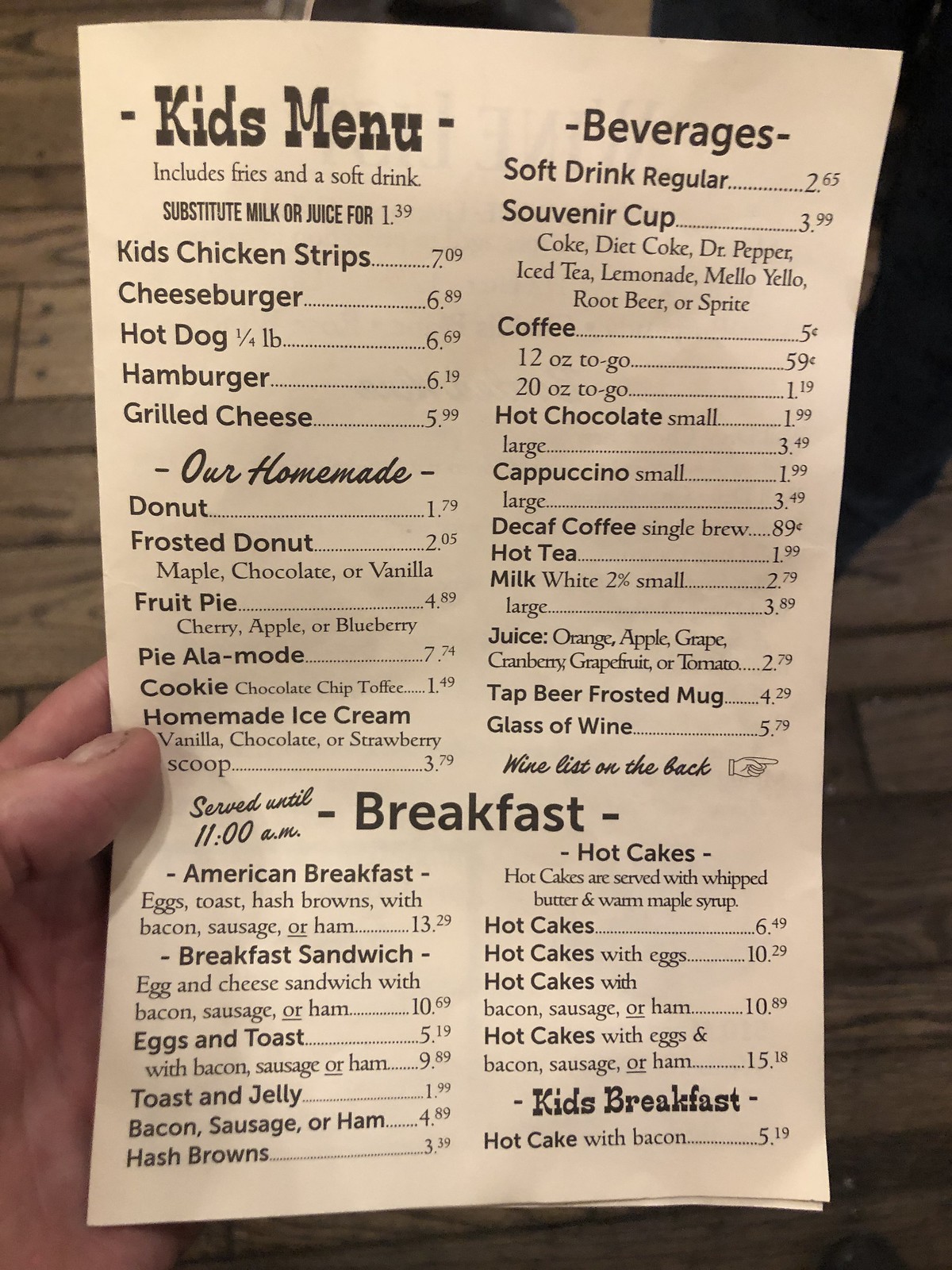In this indoor photograph captured with a regular camera, a masculine white hand is holding up a menu. The menu, printed in black letters on a beige background, is titled "Kids Menu" and includes the note "includes fries and a soft drink." The layout of the menu is well-organized, with food items listed down the left side and beverages down the right. 

For the main meal, the kids can choose from options like chicken strips, a cheeseburger, a hot dog, a hamburger, or a grilled cheese sandwich. In addition, there's a section for desserts featuring items such as a frosted donut, fruit pie, pie a la mode, a cookie, and homemade ice cream available in one scoop or more. 

The beverage section offers a variety of choices including soft drinks, available in a regular cup or a souvenir cup, as well as coffee (regular, decaf, and hot tea), hot chocolate, cappuccino (both small and large), milk, juice, tap beer served in a frosted mug, and glasses of wine. 

Towards the bottom, it mentions a "Breakfast Center" which is served until 11:00 a.m. This part of the menu includes various breakfast items, also featuring a dedicated section for kids' breakfast. All items on the menu have their respective prices listed on the right side. The image captures both the detailed design and content of the menu clearly.